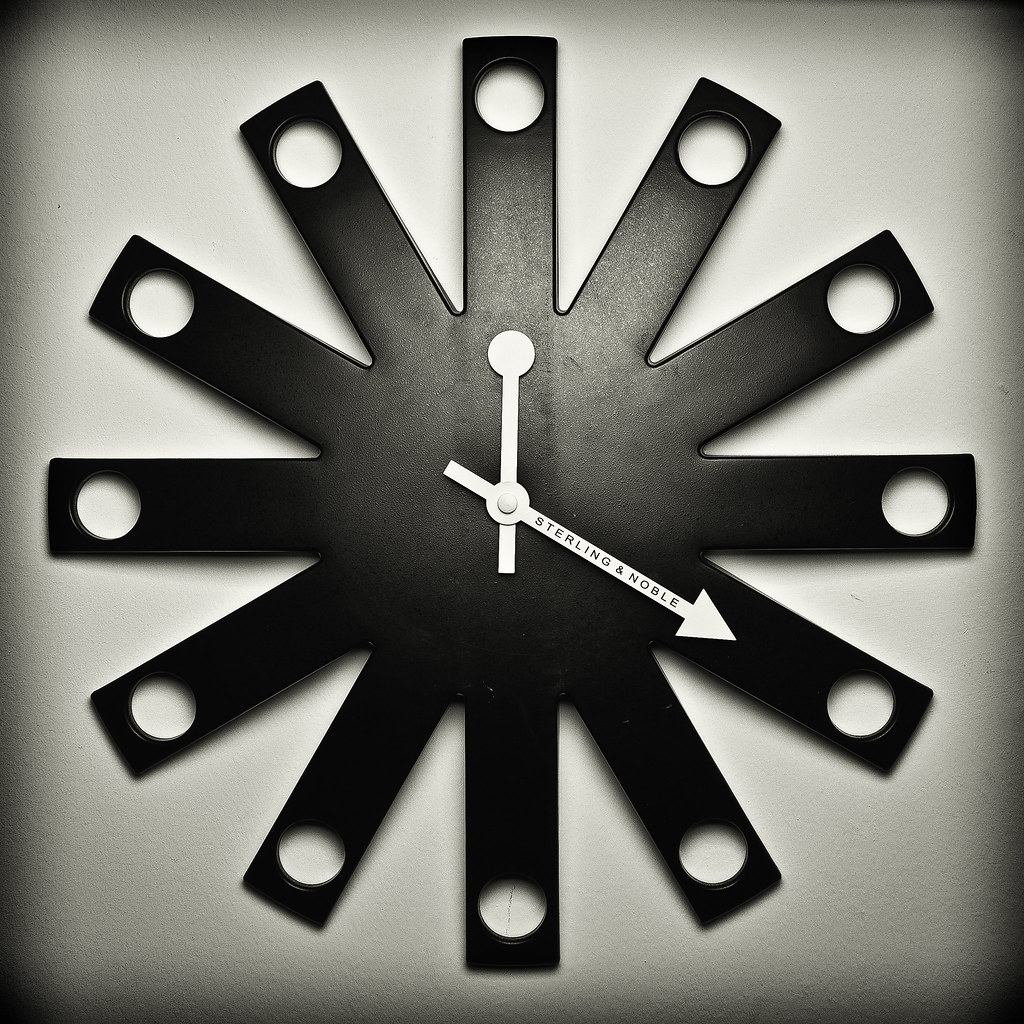This is a color photograph of an unusual, sunburst-type clock mounted on an off-white wall. The clock is predominantly black and features a distinctive starburst pattern radiating from a circular black center. The clock's starbursts are rectangular in shape, with each of the 12 serving as a marker for each hour of the day. At the end of each rectangular burst is a round, equally-sized hole, allowing the background on which the clock is mounted to show through. The design ingeniously combines black plastic or metal materials. The clock face lacks any numbers, making its sleek design even more striking. The white hands of the clock stand out prominently against the black face; the hour hand is topped with a round circle, while the minute hand has an arrow and features the black lettering "Sterling and Noble." The clock appears to indicate a time setting of about 12:20. No people are present in the image, further emphasizing the clock as the focal point.